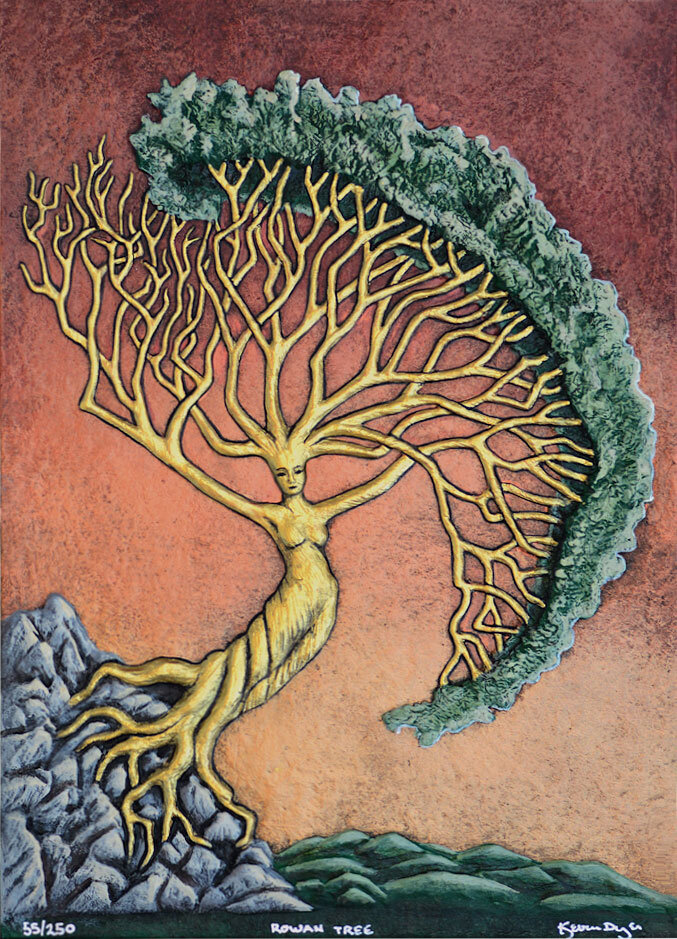This detailed painting, titled "Rowan Tree" and signed by Kevin Dreyer, is a stylized illustration numbered 55/250. The artwork features a woman seamlessly integrated into a tree, with her legs entwined as roots burrowing into a blue rock on the left and a green rock on the right. Her upper body transitions into the trunk, with visible breasts and arms outstretched, transforming into branches. Her hair also extends upwards, merging with the branches. The branches culminate in green foliage forming a large semi-circle framing her figure. Her face, bearing eyes, a nose, and a mouth, gazes forward from the tree's trunk. The background exhibits a reddish-brown hue, reminiscent of a sunset or sunrise, intensifying at the top. Additionally, there are green, rolling hills or waters in the distance, contributing to the serene and mystical ambience of the painting.